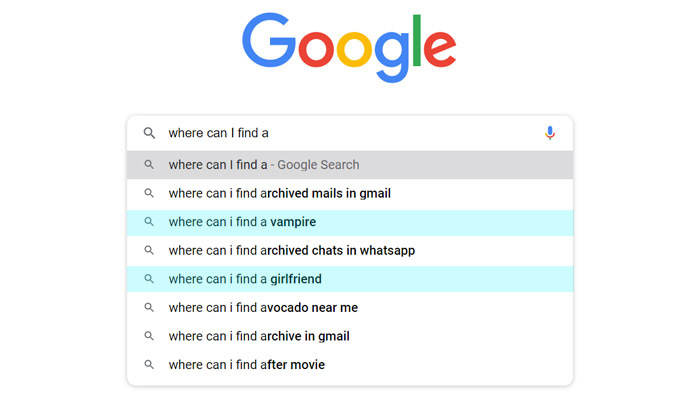The image displays a Google search interface. At the top, there's a Google logo, with each letter in its characteristic colors: a capital blue "G", followed by a lowercase red "o", a lowercase yellow "o", a lowercase blue "g", a lowercase green "l", and finally a lowercase red "e". Below the logo, there's a search bar featuring a small magnifying glass icon on the left side of the bar, and a microphone icon on the right side.

Inside the search bar, the partially typed query reads "where can I find a". A drop-down menu is expanded below the search bar, showing suggested search queries. The suggestions in the drop-down menu are as follows:

1. "where can I find - Google search"
2. "where can I find archived mails in Gmail"
3. (Highlighted in blue) "where can I find a vampire"
4. "where can I find archived chats in WhatsApp"
5. (Highlighted in blue) "where can I find a girlfriend"
6. "where can I find avocado near me"
7. "where can I find archive in Gmail"
8. "where can I find"

Each suggestion on the list is preceded by a small magnifying glass icon on the left side.